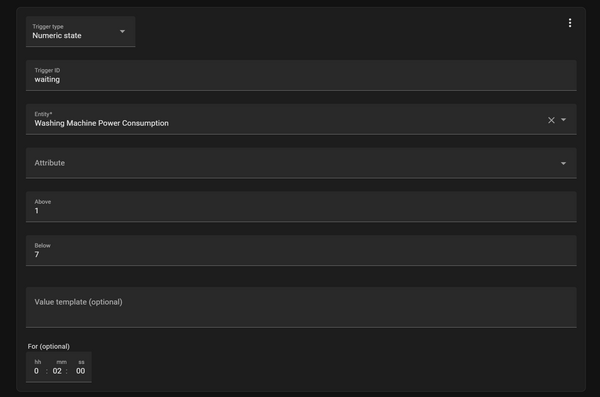A web page features a dark theme with six horizontally-aligned, lighter black boxes spanning the full width of the page. 

1. **First Box**: A short box displaying "Numeric State" with a drop-down arrow on the left and three vertical dots on the right.
2. **Second Box**: A lighter black box displays "Waiting" followed by an entry labeled "Washing Machine Power Consumption." Two icons—a crossed-out 'X' and a drop-down arrow—are on the right side.
3. **Third Box**: This box contains an "Attribute" entry with a drop-down arrow on the right.
4. **Fourth Box**: This contains an entry with the number "1" and additional unreadable text, including the number "7."
5. **Fifth Box**: Features a "Value Template" with the word "Optional" in parentheses beneath it.
6. **Sixth Box**: A short box marked "Four" with "Optional" in parentheses next to it. Below it, there appears to be a date format with the values "002" and "00."

The arrangement and details suggest this web page is possibly a form or a settings interface with various fields and options for user input.